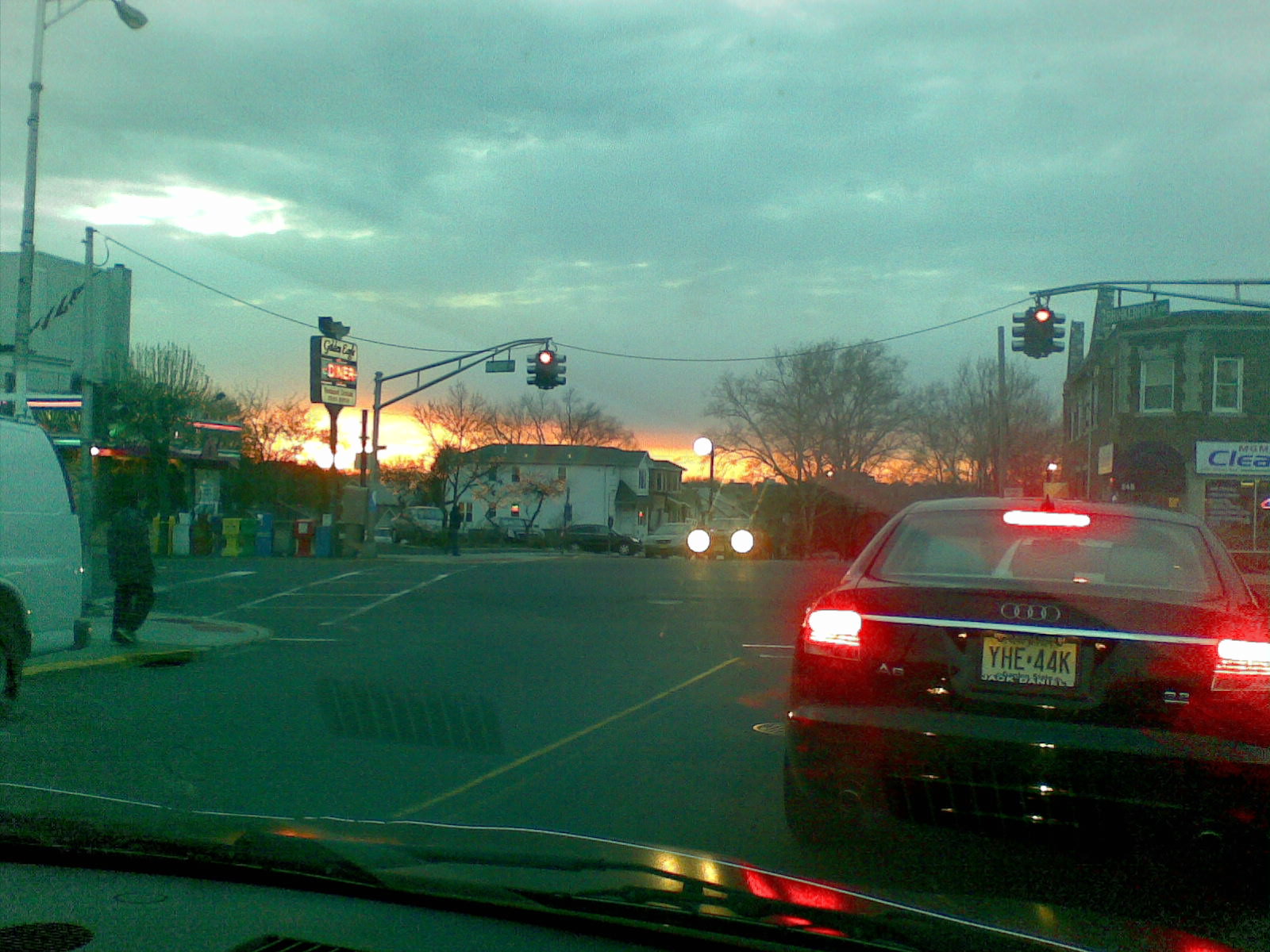As evening falls, a dark gray, cloud-covered sky stretches across the scene, highlighted by a narrow strip of bright orange along the horizon, signaling the end of the day. Tall electric lines, some touching and running horizontally, form a stark silhouette against the dimming light. Below these lines, a cylindrical black traffic light with three protruding sections displays a glowing red signal. In the distance, the word "diner" glows in red neon on a sign, adding a touch of warmth to the cool evening tones. A white house with a gray roof stands quietly further back, adding to the suburban landscape. Directly in front, a black car, its red brake lights illuminating and its license plate visible, completes the composition, capturing the tranquil yet bustling moments of the setting.